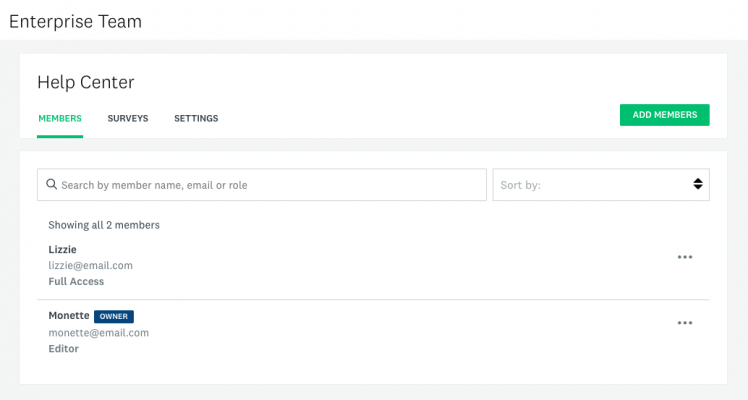This screenshot, evidently captured from a desktop or laptop computer given the UI size and widescreen landscape format, displays an interface titled "Enterprise Team." Set against a gray background, the image features several white content windows.

At the top, there is a window labeled "Help Center" which includes buttons for "Members," "Surveys," and "Settings." A prominent green "Add Members" button is located on the right side. The "Members" setting is currently selected.

Below this, another content window appears, which contains a search bar labeled "Search by member name, email, or role," accompanied by a "Sort by" dropdown menu positioned to the right. Directly beneath this, there are search results indicating two members:

1. Lizzy (lizzy@example.com) with "Full access."
2. Monette, designated as the "Owner" (monette@example.com) with "Editor" access.

Each member entry includes a "More options" button, represented by three horizontal dots to the right. This interface appears to be a setup page for a team collaboration or work portal, designed to manage and organize team members efficiently.